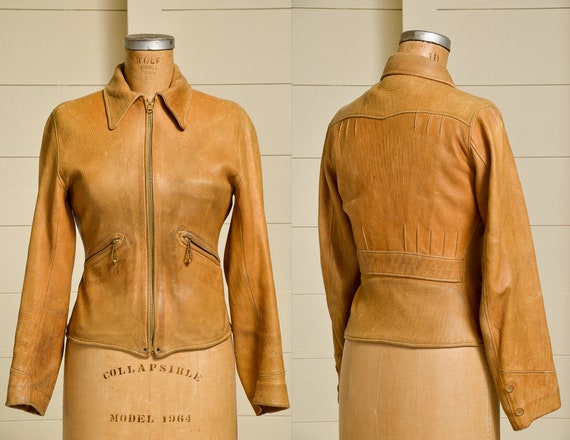A detailed image features a headless wooden mannequin displaying a stylish leather jacket. The brown leather jacket, which exhibits a blend of light orange and brown hues, is zipped up in the middle and includes notable detailing such as a collar and long sleeves. The jacket's practical design includes two zippered pockets, with one zipper running diagonally from the bottom right to the top left and the other from the bottom left to the top right. On the neck of the mannequin, text reads "Collapsible," although it's challenging to fully decipher, followed by "Model 1964." The image creatively splits the view, presenting the front of the jacket on the left half and the back on the right half, giving a comprehensive perspective of the jacket's design. The backdrop showcases white wood floors, adding an elegant contrast to the scene.